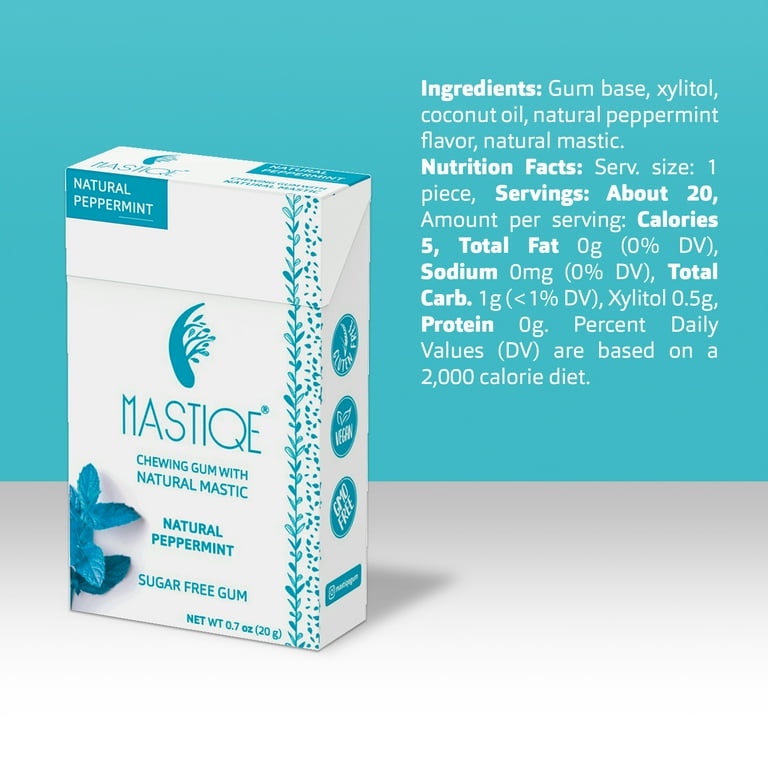This advertisement features a brand of chewing gum called "Mastique," spelled M-A-S-T-I-Q-E. The image is divided into two main sections: the upper two-thirds showcasing a bright light blue color, while the bottom portion transitions from gray to white in a gradient. On the left side of the image, a box of Mastique chewing gum is prominently displayed. The box, reminiscent of a cigarette pack, is white with turquoise blue and light blue decorations that mirror the background hues.

The Mastique branding runs across the center of the box in turquoise blue, accompanied by a stylized emblem resembling a raindrop with tree branches emerging from it. A blue-green vine illustration extends along the right side of the box from top to bottom. Below the Mastique name, the phrases "chewing gum with natural mastic," "natural peppermint," and "sugar-free gum" are clearly printed.

On the right side of the image, detailed lists of ingredients and nutrition facts are displayed in white text, resembling a typical nutrition label. The ingredients include gum base, xylitol, coconut oil, natural peppermint flavor, and natural mastic, while the nutrition facts indicate one serving contains roughly five calories, with 20 servings per box, and no fat, sodium, or protein.

Overall, the advertisement emphasizes the natural, sugar-free qualities of the Mastique peppermint chewing gum and provides comprehensive ingredient and nutritional information while maintaining a clean and appealing blue-white color scheme.